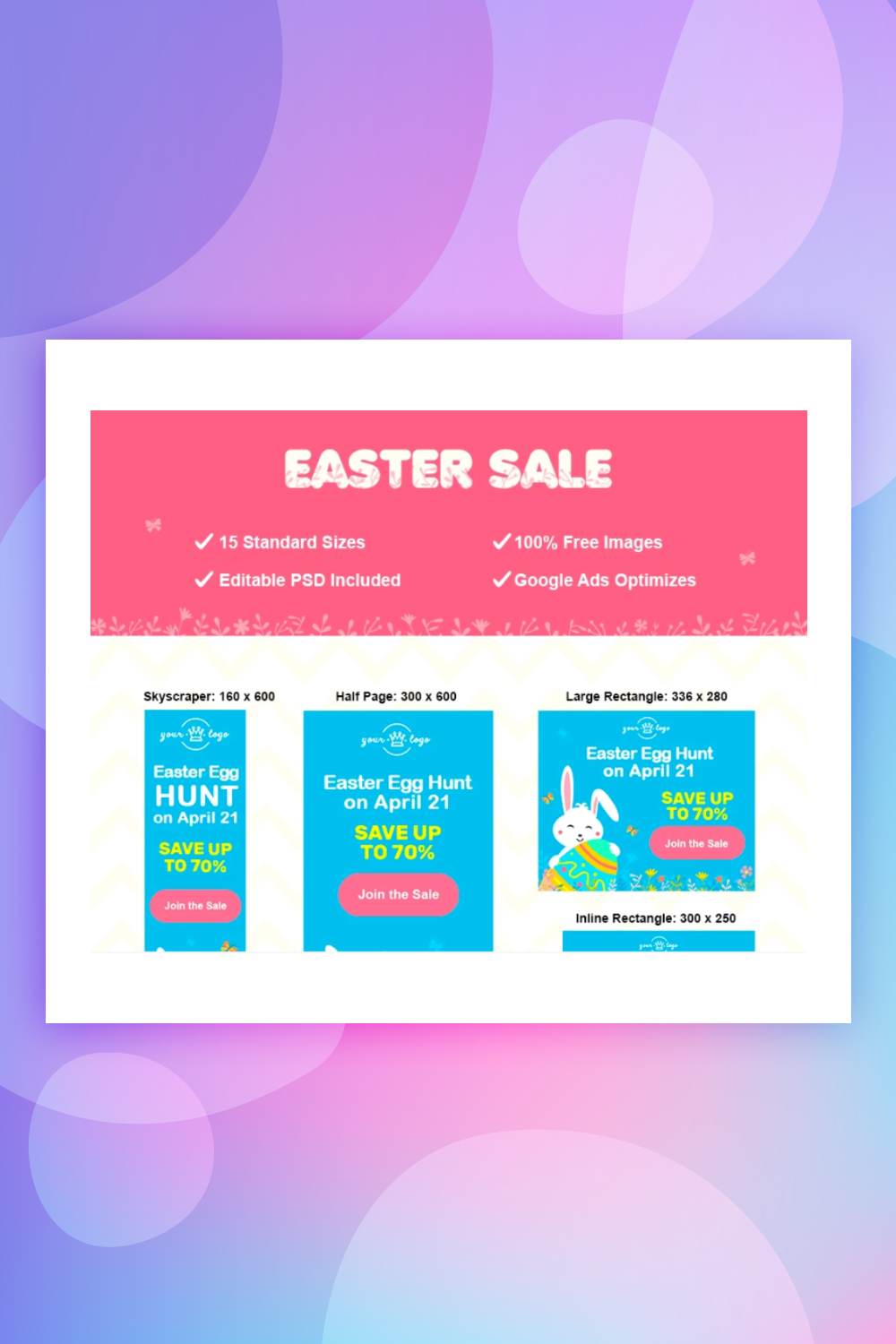The screenshot depicts a vibrant and festive Easter sale advertisement. The background showcases a palette of pastel colors, including shades of purple, lavender, lighter purple, light blue, and medium blue. Overlaying the background are various translucent ovals and blobby circles, which are stacked and floating, creating a visually appealing and layered effect.

At the center of the image, a white floating field with a soft drop shadow serves as the main focus. This field is topped with a prominent pink header bordered in white. The words “Easter Sale” are displayed in playful bubble letters, adorned with delicate pink branches or twigs partially overlaying the bottom halves of the letters.

Below the headline, four check-marked features are listed:
1. 15 Standard Sizes
2. Editable PSD Included
3. 100 Free Images
4. Google Ad Optimized

The lower part of the ad features additional plant graphics and butterflies, enhancing the Easter theme. 

Beneath this, the layout includes various fields likely indicating different ad mock-ups. The first field, labeled "skyscraper, 160 by 600," promotes a "Blue Easter Egg Hunt on April 21st" with savings of up to 70% and an invitation to join the sale. The "half page, 300 by 600" field contains the same information but with wider spacing.

The "large rectangle, 336 by 280" also repeats the sale details but is complemented by illustrations of an Easter bunny and an egg positioned on the left side. Additionally, the field labeled "inline rectangle, 300 by 250" appears below but is cut off in the screenshot.